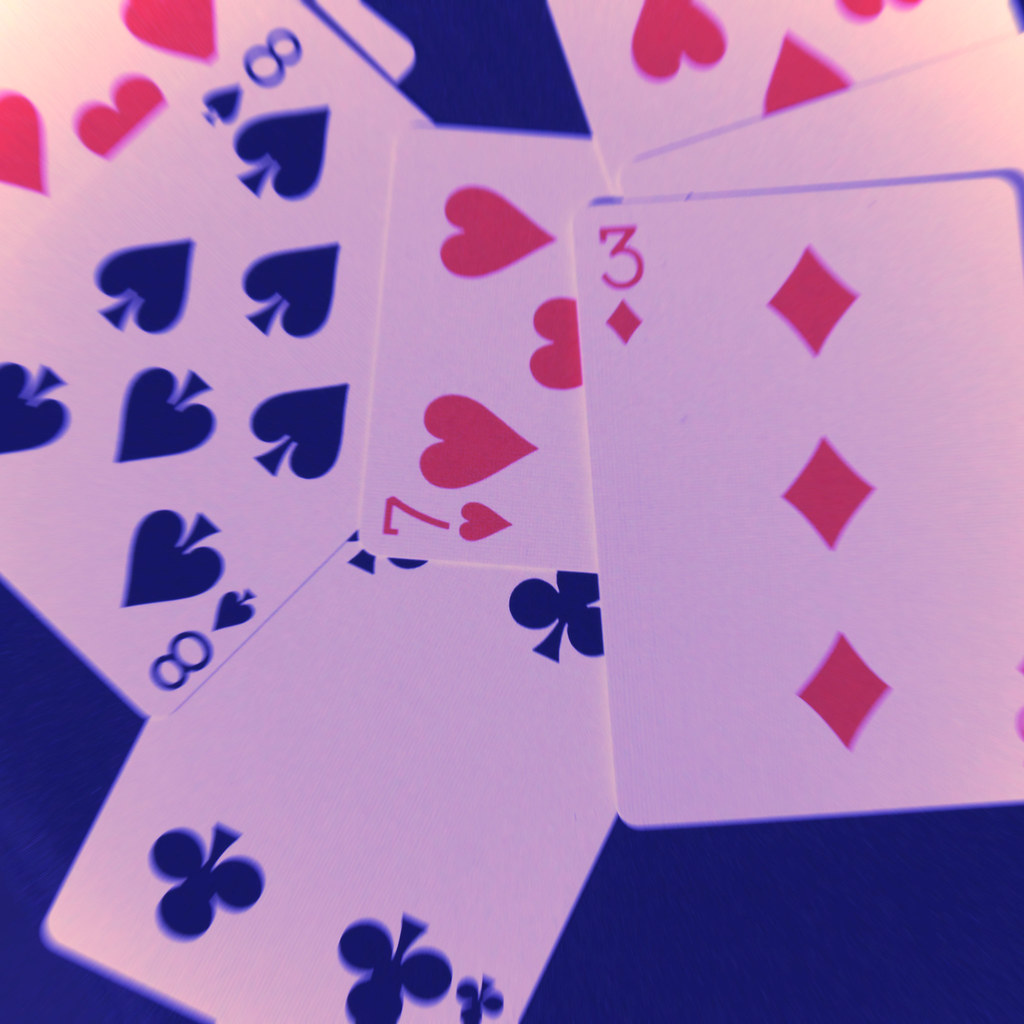The image showcases a pile of playing cards set against a royal blue background. Prominently displayed at the top of the pile is a three of diamonds; the card's white face is contrasted by its red diamond symbols, centrally located within the frame. Positioned to the left of the three of diamonds and partially overlapping it is a seven of hearts, distinguishable by its red heart symbols. Beneath the seven of hearts, in the upper left-hand portion of the image, lies an eight of spades, marked by black spade symbols. Some parts of the eight of spades, specifically the upper right-hand and lower left-hand corners, are obscured by the overlapping seven of hearts card. Additionally, there appears to be a few more cards in the pile, including what seems to be a four of clubs at the bottom, although its exact number is somewhat uncertain as it is partially out of the frame.